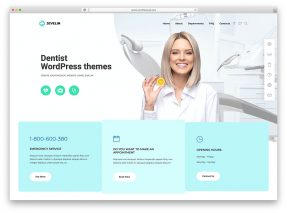The image depicts a low-resolution website with a primarily white background, accented with green and black. The site features a header that reads "Dentist WordPress Themes." At the center of the image stands a woman with shoulder-length, straight blonde hair that is darker at the roots. She is holding an indeterminate yellow object. Behind her is a white dentist chair, set within a typical white-walled dental clinic environment.

At the bottom of the image, there are three turquoise-colored boxes, each displaying a distinct icon and black text beneath them. The leftmost box features a black-font 1-800 number. The middle box likely has a calendar icon, while the rightmost box displays a clock icon, both also with black text underneath. Each box includes a white button, though the text on them is unreadable due to the image's poor resolution.

Overall, the website features a palette that includes black, white, various shades of turquoise, gray, a peachy tan, red, yellow, green, and the woman's multi-tonal blonde hair. The URL bar is visible but illegible, contributing further to the general lack of clarity in the image.